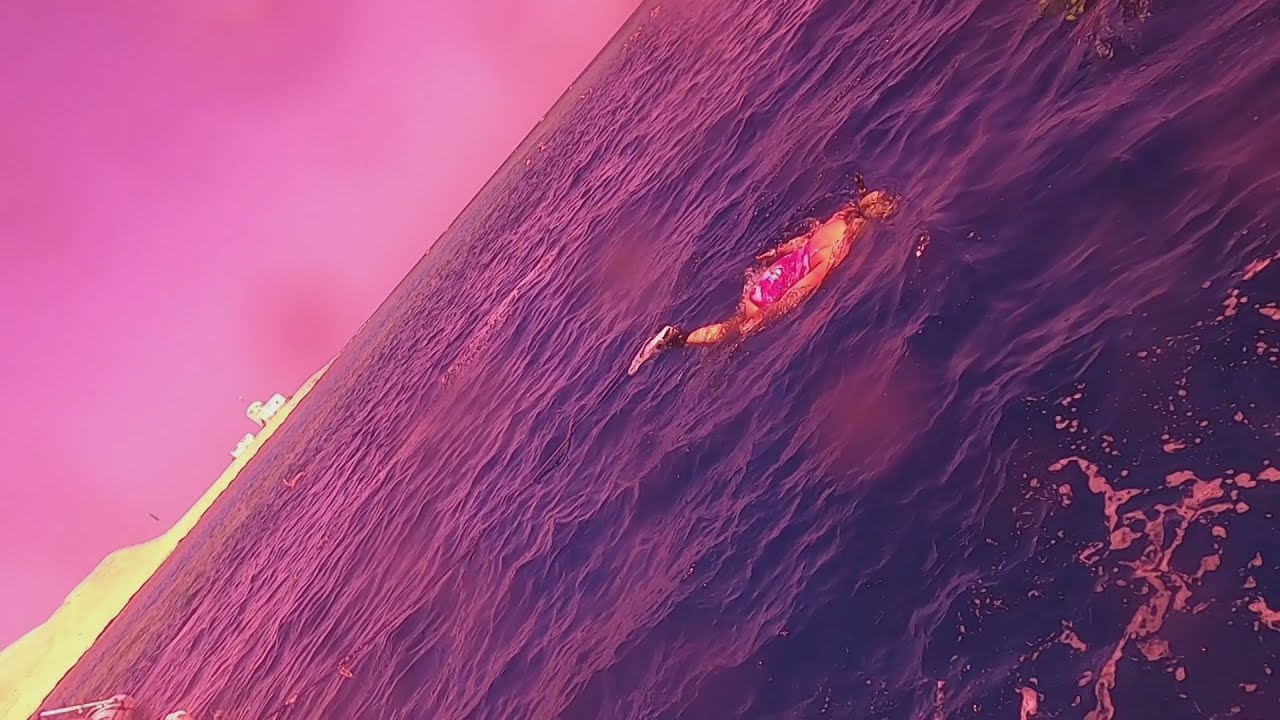This horizontally aligned, slightly tilted rectangular photograph captures a tranquil scene bathed in hues of purple. The sky, cloaked in a blend of light and dark purples, spans the upper left to the bottom left of the image, creating an ethereal atmosphere. The rest of the scene is dominated by the ocean, which mirrors the sky’s purplish-blue tones. Diagonally set, the picture gives a unique perspective on the serene seascape.

Central to the image is a lone swimmer, likely a female, engaged in snorkeling. Her body is flat against the water’s surface, head submerged, and only her back visible, adorned in a pink and white patterned swimsuit. One of her black fins is prominently raised above the water, adding to the dynamic feel of her motion.

In the background, at the border where the sky meets the water on the lower left corner, a white structure resembling a building stands on an irregularly shaped land form or hill, tinged in desert dune colors. This element adds a hint of terrestrial connection to the otherwise aquatic and open scene. The overall composition, with its slanted alignment and vivid purples, gives the photograph an artistic and dreamlike quality, emphasizing the solitary swimmer amidst the expansive, colorful seascape.